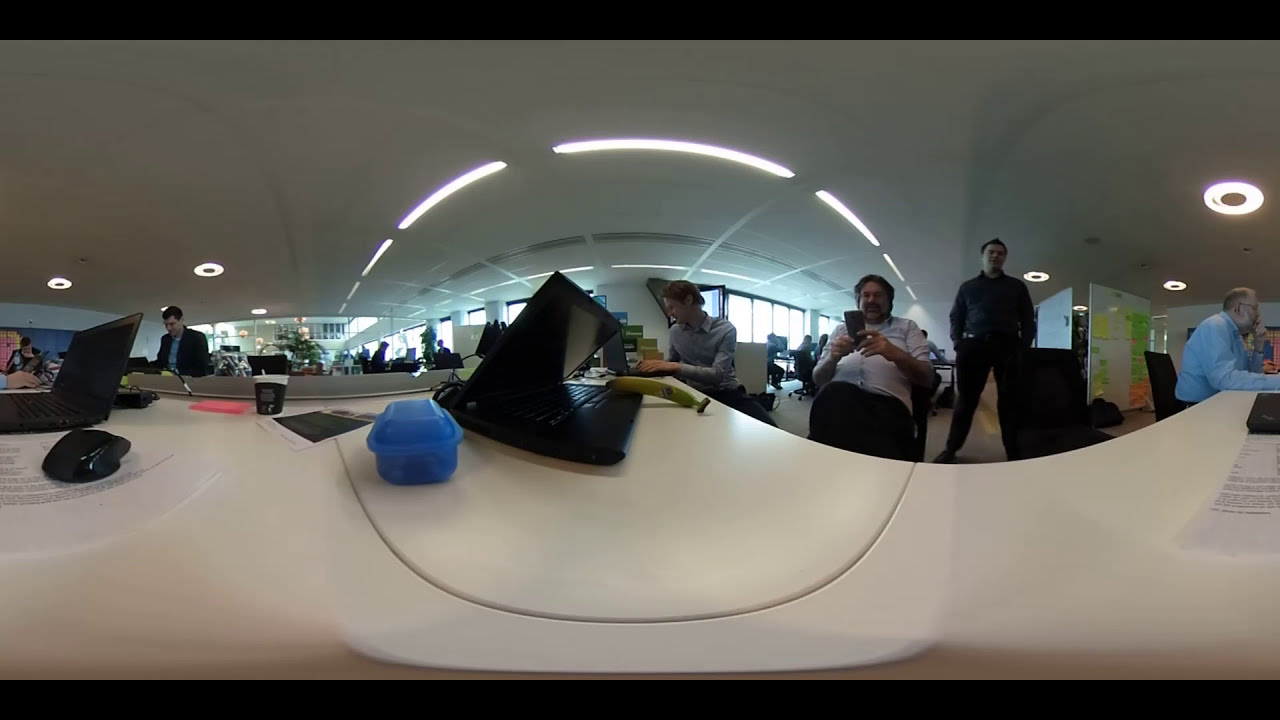In a panoramic 360-degree shot of a modern, curved office space, the scene captures a bustling work environment. At the center, a sleek, large white table dominates the room, stretching from the right to the left and adorned with various laptops, including one notably with a banana on it. Five gentlemen are engaged in different activities around the table. One man, somewhat older and heavier, leans back in his chair, engrossed in his cell phone, while the skinnier man next to him focuses on his laptop. Another middle-aged man stands behind them, dressed in all black with hands in his pockets, observing the scene. To the backdrop of this central activity, multiple other individuals are visible, diligently working across the stylish white curved desks that contour dips and rises, reflecting light and shadow.

Along the wall of the office, a series of curved windows allows natural light to stream in, enhancing the vibrant atmosphere. A small blue tote and various office supplies are scattered across the surface of the white table. On the right side of the image, a large map and whiteboards with papers taped to them provide evidence of ongoing projects and brainstorming sessions. The rounded ceiling, painted a pristine white, features arched, rainbow-shaped lights and circular fixtures that add a modern touch to this dynamic workspace. In the distance, the atrium space is visible, further emphasizing the expansive and open design of this lively office environment.